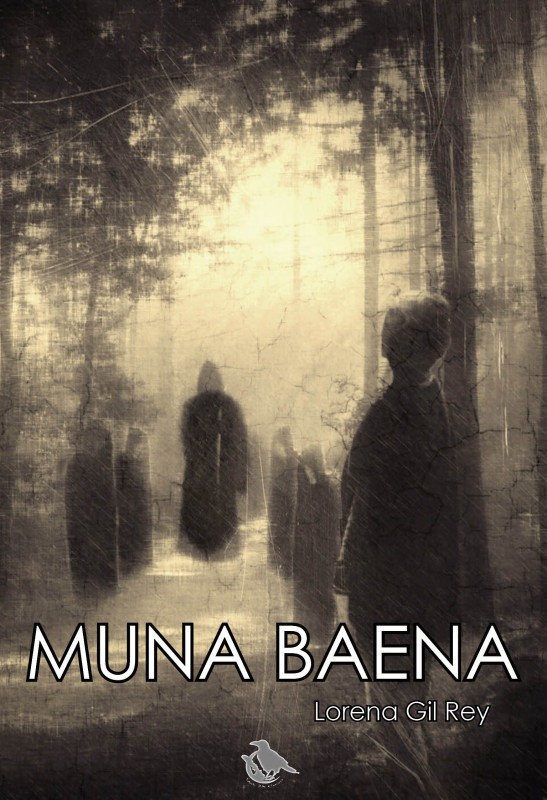This sepia-toned, slightly blurry image with hints of black and white and a brownish cast, appears to be a book cover for the title "Muna Baena" by Lorena Gilray. The setting is a spooky forest where tall, skinny trees create a canopy overhead. In the center of the image, a hooded character dressed in a dark cloak walks away into a bright yellow light, framed by two cloaked figures on each side who seem to watch them. Closer to the foreground, another robed figure with either white hair or a white cap stands watch, adding to the eerie atmosphere of the scene. The bottom of the image features the title "Muna Baena" in large white font with "Lorena Gilray" beneath it, and a small logo depicting a crow perched on a moon, further contributing to the ghostly, esoteric feel of the cover.